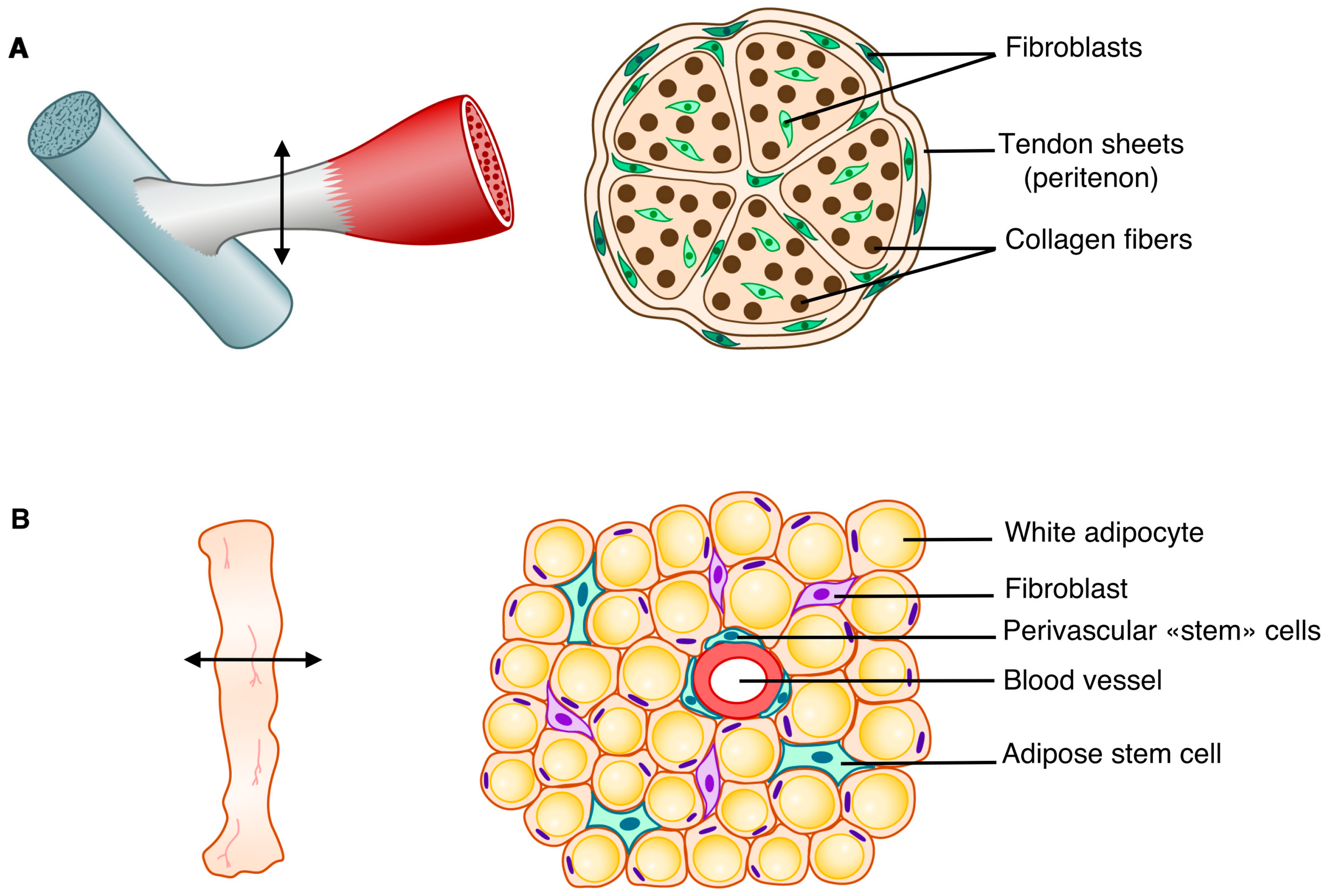This image features four diagrams labeled A and B, reminiscent of illustrations from a medical textbook. Each label contains two images, presenting a detailed examination of anatomical structures possibly related to tendons and fat cells. In Image A, the first diagram depicts a structure resembling a chicken leg extending from a metal pole. Adjacent to it is a detailed cross-section, labeled to identify various internal components such as green fibroblasts, brown collagen fibers, and tendon sheaths. The second diagram in Image A lays out these elements more intricately, resembling a T-bone shape with blue, white, and red hues suggesting blood vessels.

Image B contrasts with a different focus, possibly representing a human leg or an unusual form thereof. Its diagrams feature cross-sections labeled with white adipocytes, fibroblasts, perivascular stem cells, blood vessels, and adipose stem cells. The representation also includes an illustration that appears bone-like, depicted in tan with directional arrows for clarity. This detailed presentation aims to educate on the intricate inner workings of tendons and fat cell structures, marked with precise labels to differentiate between various cellular components and tissue types.